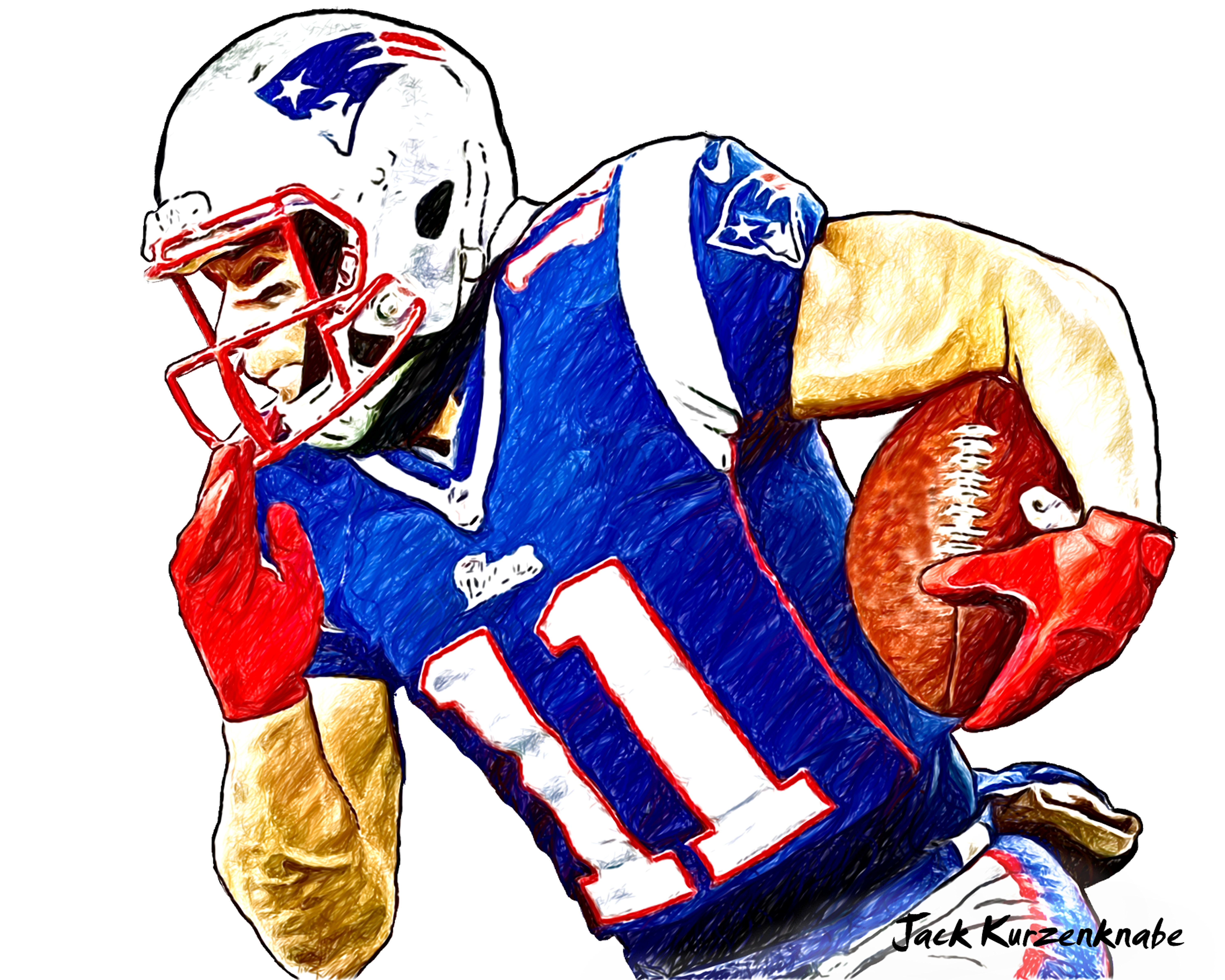This detailed and realistic digital art piece, signed by artist Jack Kurzenabe, portrays Julian Edelman, the New England Patriots' number 11. The quarterback is captured mid-run, displaying a dynamic sense of motion, moving from right to left. He dons a blue jersey with the number 11 prominently featured in white text with a red border. Complementing his attire, Edelman is adorned in white pants with red and blue stripes, red gloves, and a distinctive silver helmet bearing the Patriots' emblem. The helmet's visor is accentuated with red bars. Edelman's right arm is bent, his right hand almost touching his helmet, while he carries the football securely in his left arm. A hand-warming pouch is noticeable, twisted around to rest on his lower back. The artist's signature, "Jack Kurzenabe," is displayed in black text on the bottom right corner of the image, underscoring the authenticity and attention to detail in this digital masterpiece.